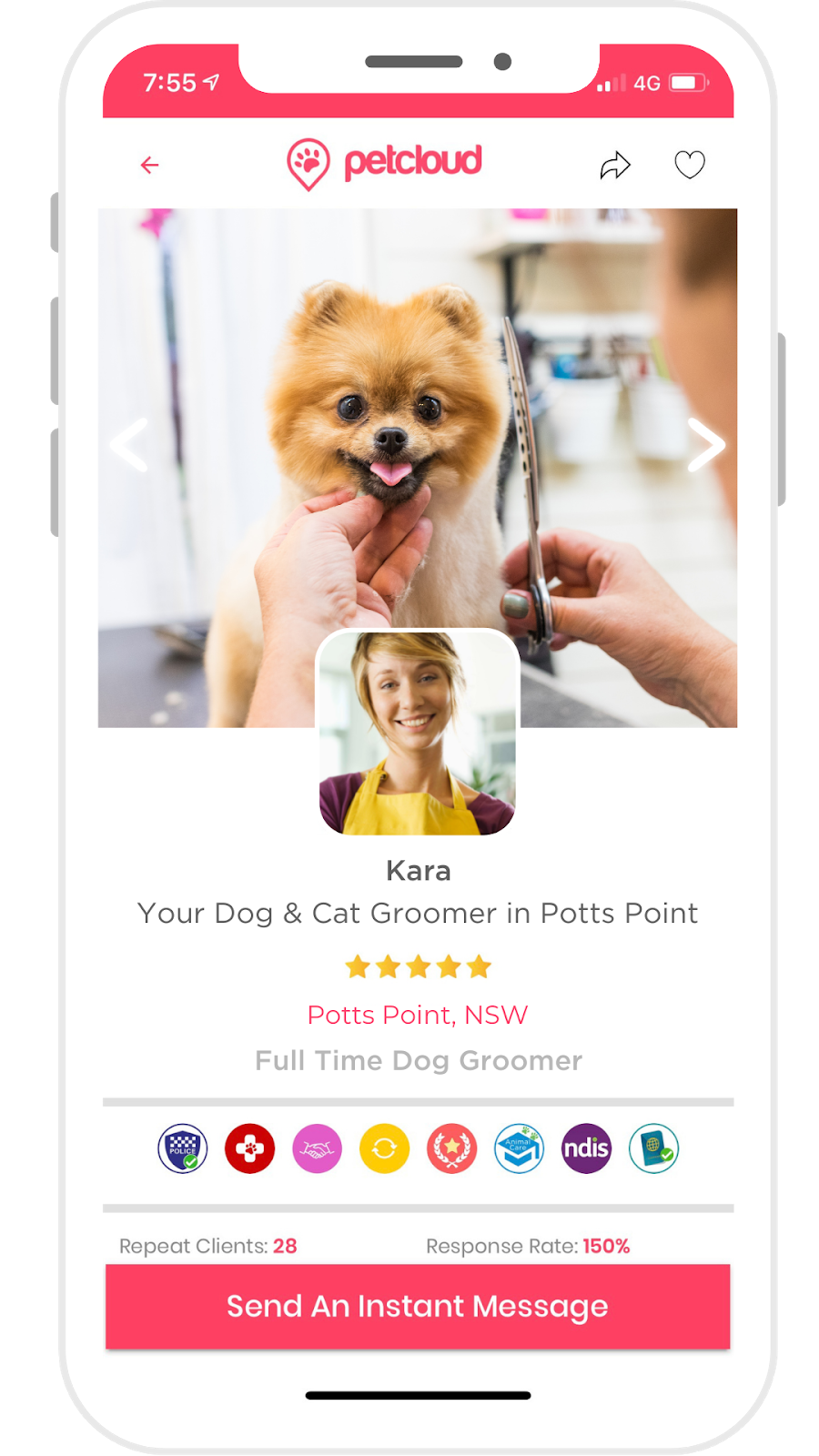In this image, we see a smartphone displaying an app named "PetCloud." The app interface features a predominantly white background with accents of a pinkish-red color. At the top of the screen, the PetCloud logo is prominently displayed alongside a return button, a heart icon, and a circular icon depicting a dog's paw.

Further down the screen, there is a photograph of a small, light golden-brown dog, reminiscent of a golden retriever's coloring. The dog appears to be in the midst of a grooming session, as a person, either a man or a woman, is shown trimming the dog's hair.

Below this image, we see a portrait of a woman named Kara, identified as "Your dog and cat groomer in Potts Point." Kara's profile is highlighted by a five-star rating, suggesting a high level of customer satisfaction. Her profile indicates that she is a full-time groomer, and beneath her title, several emblems are displayed, possibly signifying various certifications or achievements.

At the bottom of the screen, additional statistics are presented: Kara has 28 repeat clients, and her response rate stands at an impressive 150%. To the right of these stats, a large button invites users to "Send an Instant Message," facilitating direct communication with the groomer.